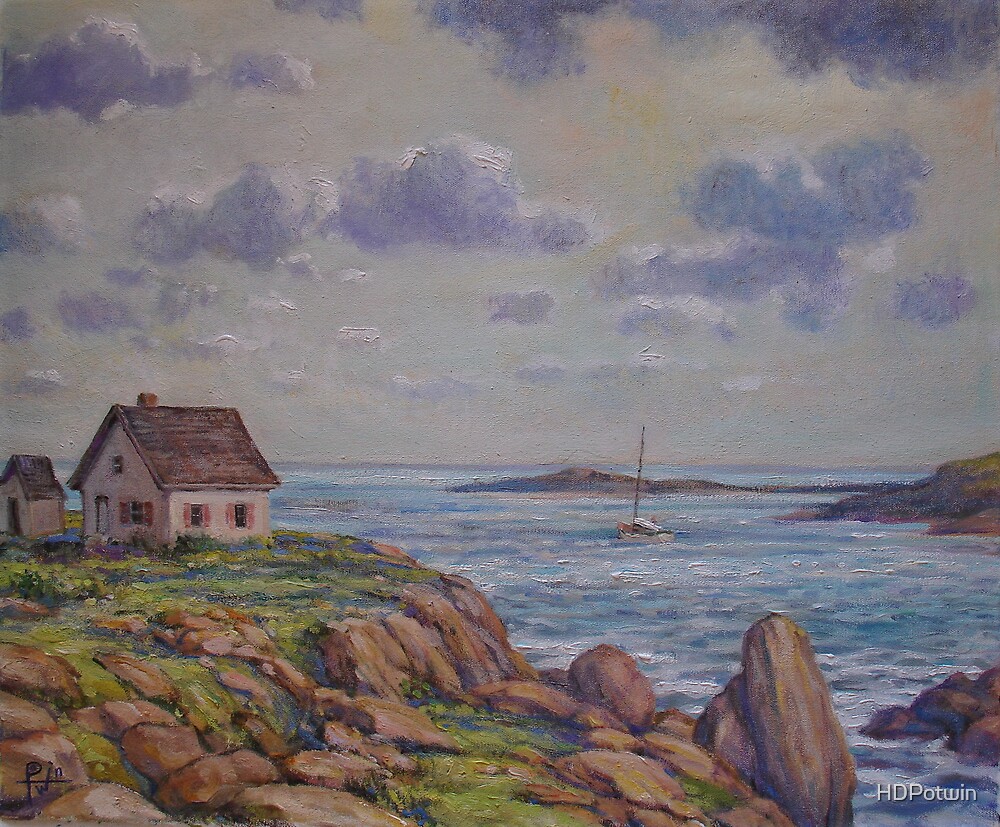This painting depicts a dramatic seascape featuring a rugged, rocky shoreline juxtaposed with a modest homestead. The central focus of the image is the small house perched on a grassy embankment. The house is painted in a light cream or dull gray color with a sloped dark brown roof and maroon shutters adorning its windows. A smaller shed or outhouse accompanies the house, sharing the same color scheme. The rocky shore below consists of large, jagged stones interspersed with patches of green grass and a few flowers.

The scene is set against an overcast sky filled with gray and light purple clouds, hinting at an impending storm. The ocean, depicted in teal hues, appears choppy with pronounced waves. A sailboat, with its sail not raised, is visible on the water, seemingly approaching the shore. 

This meticulously detailed landscape is signed "HD Potwin" in black text at the bottom left corner and features a watermark with the same name in white text at the bottom right corner, adding an air of authenticity to the artwork.